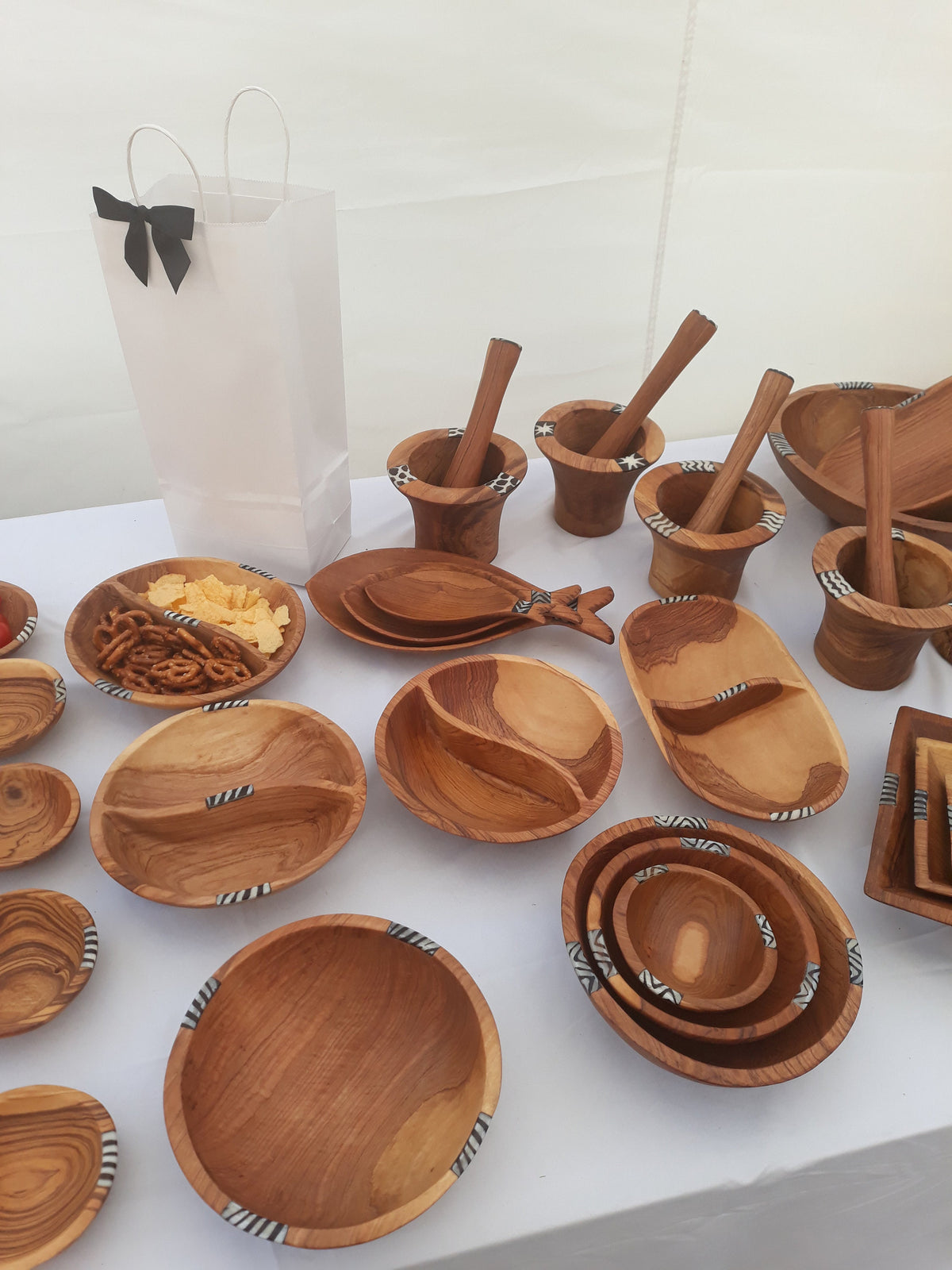This indoor photograph captures a beautifully arranged display of wooden bowls and dishes set upon a rectangular table draped in a white tablecloth. The backdrop is a white wall, possibly part of a tent, creating a clean and minimalist setting. Central to the arrangement are a variety of handcrafted wooden bowls, some plain and others intricately designed with sections. Notably, one divided bowl is filled with pretzels on one side and potato chips on the other. Beside it, a charming arrangement of three nested fish-shaped bowls adds visual interest. Additional bowls, varying from circular to square, fill the table, with some stacked neatly inside each other. Four wooden mortar and pestles with accompanying sticks are positioned in the back right corner, suggesting a multi-purpose use for grinding. A distinctive white paper bag with a black bow stands out amidst the wooden items. Decorative black and white striped patterns embellish the rims and central quadrants of several bowls, evoking an African-inspired aesthetic. The cohesive arrangement and attention to detail make for a visually appealing and intriguing photograph.